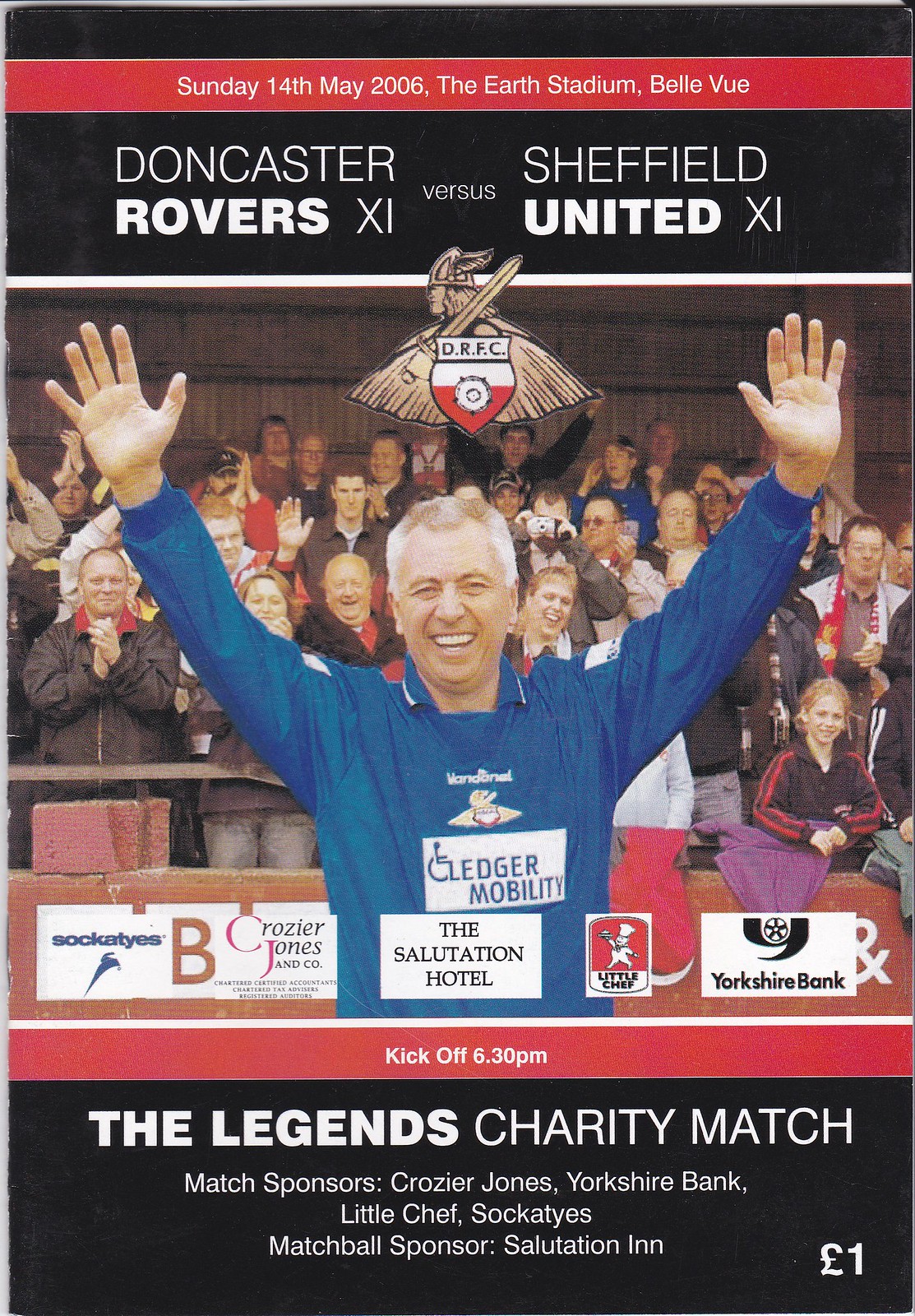A detailed poster for a charity match between the Doncaster Rovers XI and Sheffield United XI. The event takes place on Sunday, 14th May 2006, at the Earth Stadium, Bellevue, with kickoff at 6:30 PM. The top of the poster features a red stripe on a black border with white text providing the date and venue information. Below, white text on a black background announces the teams. Central to the poster is an image of a man wearing a blue long sleeve shirt with an insignia and the text "Ledger Mobility" on it, raising his hands, with a cheering crowd in the background. Above the man is a brown shield-like logo, possibly depicting an animal head. Several advertisement boxes below include sponsors such as the Salutation Hotel, Crosier Jones, and Yorkshire Bank. The bottom red strip reiterates the kickoff time, followed by another black border listing the Legends Charity Match and its sponsors. The bottom right corner displays a British pound symbol and the number 1, indicating the price. The poster's design emphasizes the charity nature of the match and its various sponsors, creating an organized promotional display for the event.